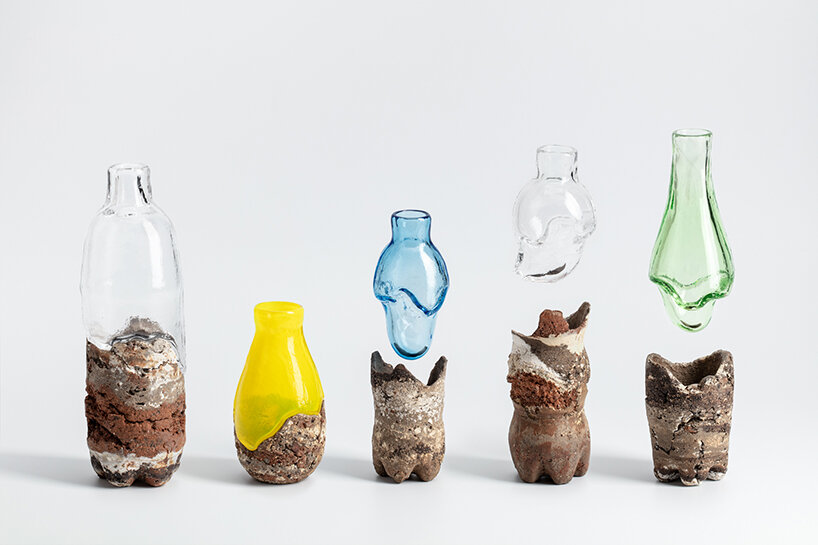This photograph captures an art piece featuring five handmade glass and stone bottle-like sculptures arranged side by side against a white background. Each sculpture consists of a distinct glass top piece suspended above a base made of red-brown clay or rock. Starting from the left, the first clear glass bottle contains carefully layered red dirt and white to pale gray stones. The second is a shorter, broken-topped bottle with yellow glass or plastic, inset onto its red-brown clay base. The third sculpture features a blue, water bottle-like glass seemingly hovering above a similar earthy foundation. Next is a sculpture with a white glass bottle hovering midair, again with the same grounded clay bottom. Lastly, the final piece displays a pale green glass bottle that resembles the silhouette of a beer bottle, also hovering above its clay base. The deliberate suspension of the glass pieces over their bases lends an intriguing, almost impossible appearance, showcasing the artist's skill and creativity.